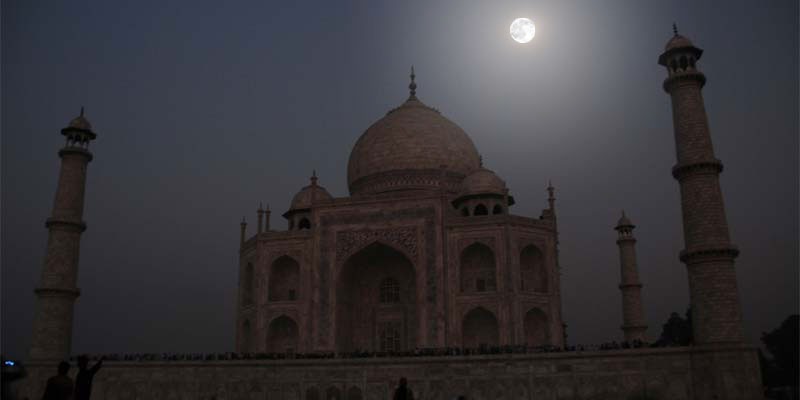The nighttime scene presents a majestic structure, likely a mosque, characterized by its distinctly foreign architectural features. The moon, prominent despite its relatively small size in the image, hangs near the top right, casting a subdued light over the scene. This illumination is the only source of light, emphasizing the silhouette of the ancient-looking structure. The central building, crowned with a large dome, is surrounded by multiple towering minarets with pointed tops, reminiscent of lighthouses. Captured from a low angle, the image highlights the building's base and intricate arches, shrouded in darkness. The structure bears a resemblance to the Taj Mahal, though it is likely smaller. The scene's stark contrast between the dark sky and the gently lit mosque evokes an aura of serene, timeless beauty.